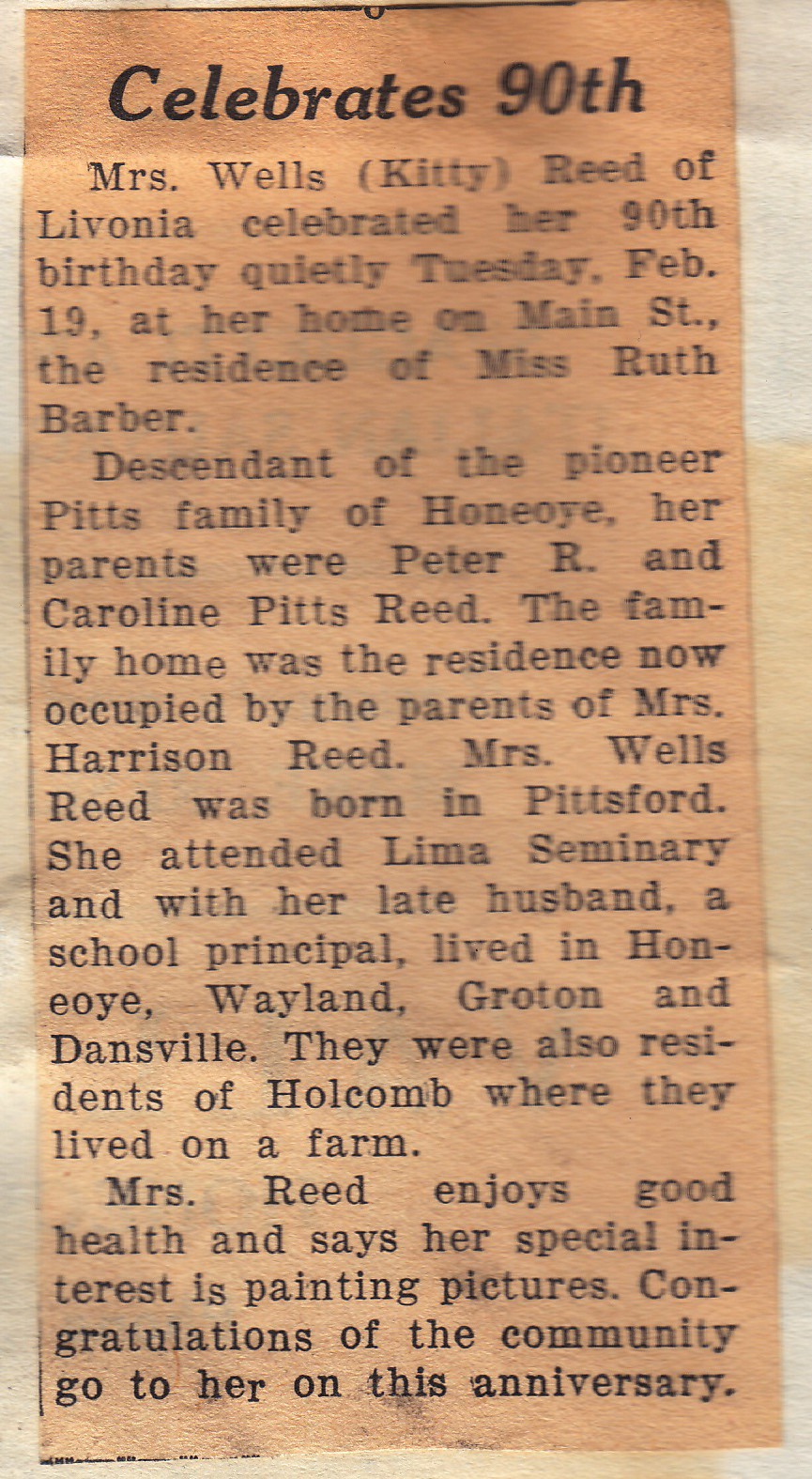The image is a black-and-white newspaper clipping with a reddish-orange hue, headlined "Celebrates 90th." The article announces that Mrs. Wells, also known as Kitty Reed, of Livonia, celebrated her 90th birthday quietly on Tuesday, February 19th, at her home on Main Street, the residence of Miss Ruth Barber. She is a descendant of the Pioneer Pitts family of Honiore (occasionally referred to as Ponyo Way or Honeyor), with her parents being Peter R. and Caroline Pitts Reed. The family home is now the residence of Mrs. Harrison Reed's parents. Mrs. Wells Reed was born in Pittsford and attended Lima Seminary. She and her late husband, a school principal, resided in places such as Hanoi, Weyland, Groton, and Dansville before settling in Holcomb, where they enjoyed life on a farm. Mrs. Reed is in good health and expresses a special interest in painting pictures. The community extends congratulations to her on this remarkable milestone.